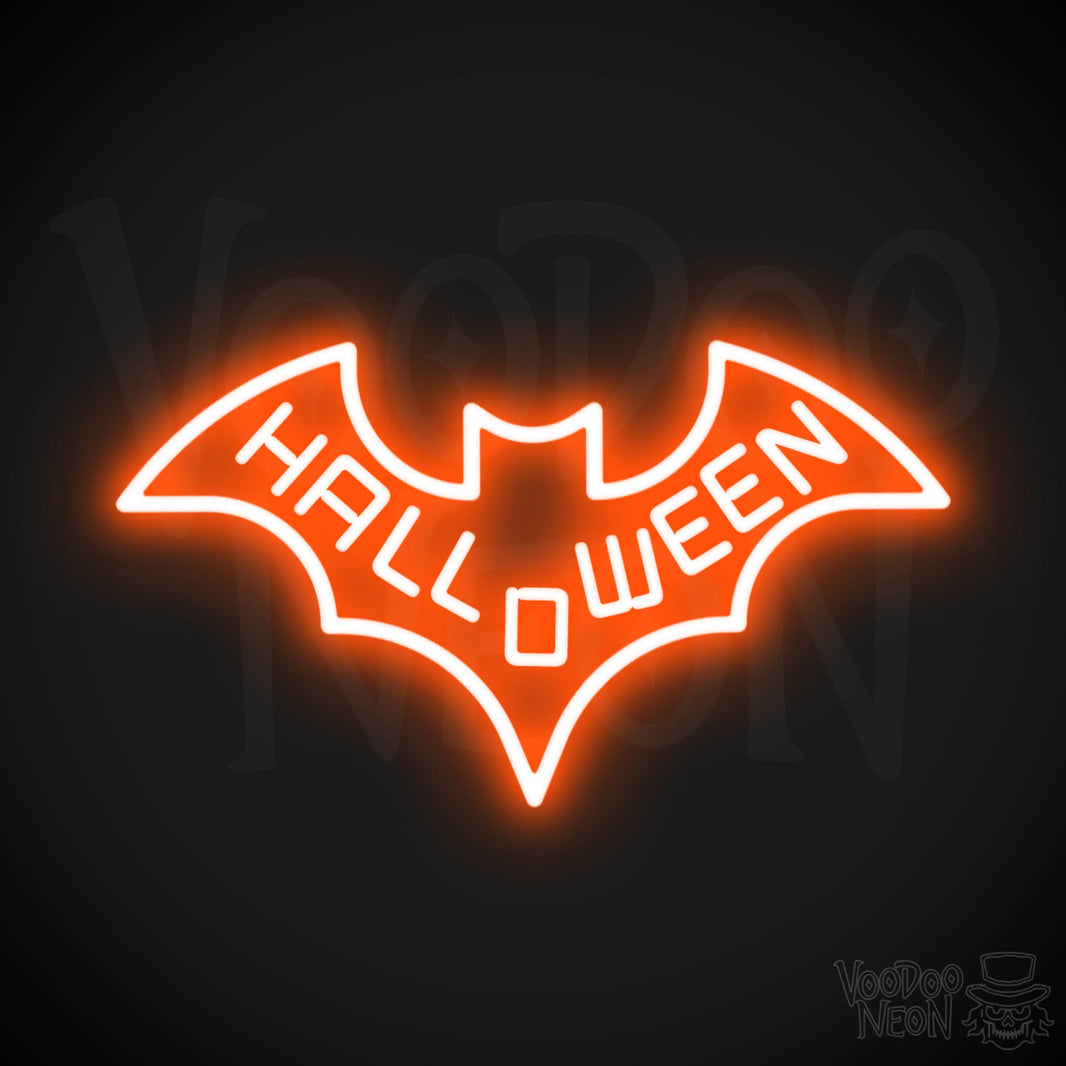The advertisement features a dramatic neon sign design set against a very dark grey or black background. Dominating the image is an orange neon bat outlined in white, with its outstretched wings displaying the word "HALLOWEEN" in all-capital, block white letters. The text spans from the upper left wing to the upper right wing, creating a striking visual effect similar to the Batman logo. Beneath this vibrant image, the company's name "Voodoo Neon" is subtly incorporated in black letters outlined in white, accompanied by a distinctive skeleton face wearing a top hat and sporting long hair. Faintly visible behind the bat is the text "VOODOO MOON," adding a mysterious layer to the dark background. The combination of eerie Halloween imagery and bold neon elements makes the ad both eye-catching and atmospheric.